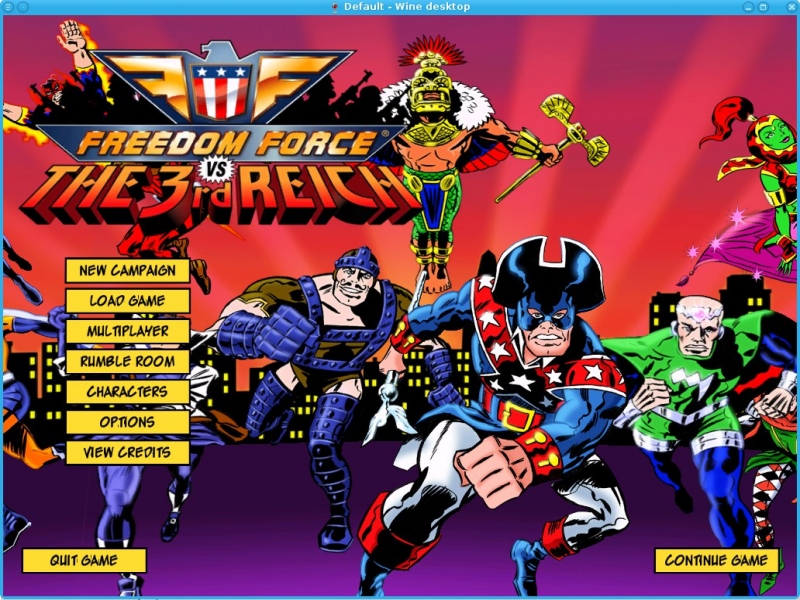The image appears to be a screenshot from a line emulator, specifically depicting the main menu of a game. At the very top of the screen, a light bar with dots is visible, along with the default line desktop interface. In the top-right corner, a small, square icon is present, while the central focus of the image is in the top-left quadrant.

The primary graphic of the game menu features an intricate design with a yellow shield resembling an American flag ornately adorned with an eagle and stretched golden wings. The text "Freedom vs. the Third Reich" is prominently displayed within the yellow shield graphic. The phrase "Freedom" is followed by "vs. the Third Reich" in substantially larger letters.

Below this, a yellow rectangular menu with black text presents various game options. The menu items listed include "New Campaign," "Load Game," "Multiplayer," "Rumble Room," "Characters," "Opera Runs," and "View Credits." The bottom-left corner of the menu shows "Quit Game," while "Continue Game" is shown to the right.

The background of the menu features dynamic rays of purple and red, creating a dramatic effect. Numerous characters are illustrated in the background. On the far right, one character stands out with exposed abdominal muscles, wielding a yellow staff and wearing a helmet adorned with a red feather. To her left stands a woman dressed in green. Below this, a man in a blue outfit, complete with a helmet, appears to the right, alongside another man donned in a green and blue-tights ensemble. Additionally, another hero clad in blue armor with a blue shield guarding his legs can be seen. The image overall showcases a lively and detailed cast of characters, emphasizing the heroic theme of the game.